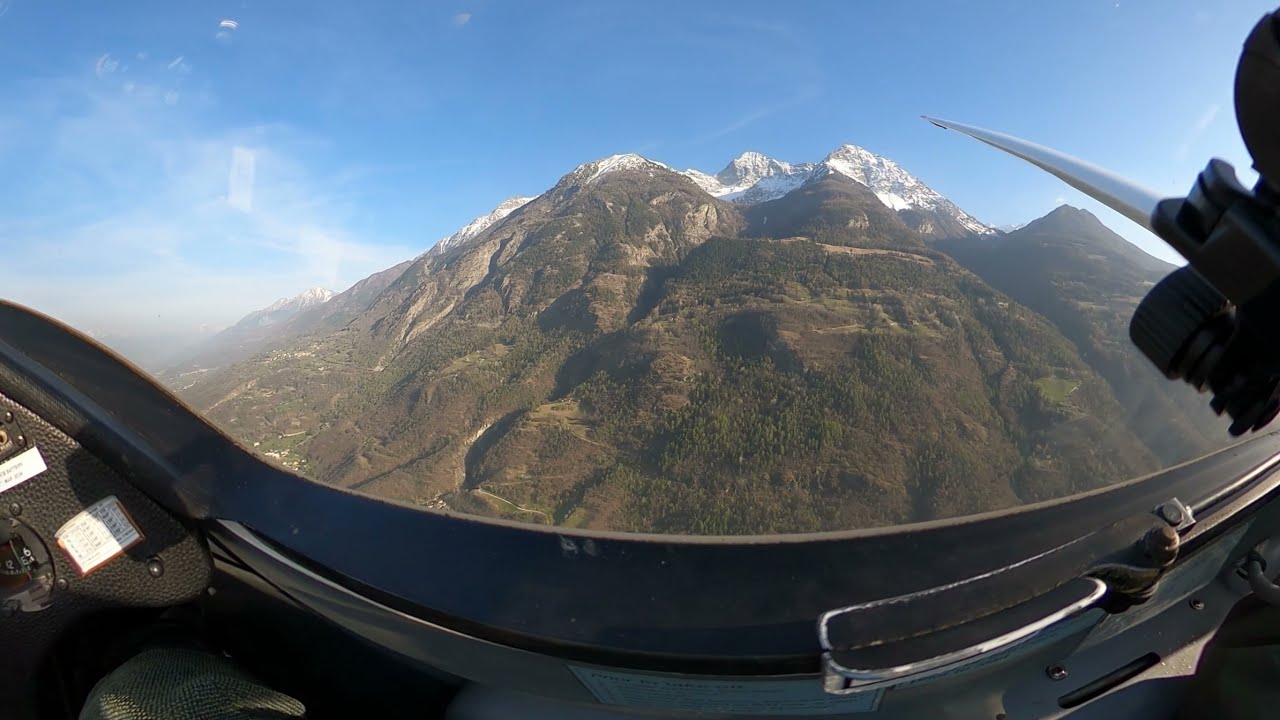The image captures the exhilarating view from the cockpit of a small, propeller-driven plane with a bubble-type canopy, flying over a majestic mountain range during a clear daytime. The photo, taken from the perspective of the pilot, reveals a sweeping panorama of the landscape below. The dominant feature is a colossal mountain, its lower slopes covered in verdant forests that transition into patches of brown and, ultimately, a snow-capped peak. Blue skies dominate the horizon with a few wisps of clouds on the left-hand side, complementing the bright and sunny ambiance, suggesting that the sun is illuminating the scene from behind the plane. Inside the black cockpit, you notice some writing and lettering, a canopy release handle positioned centrally, and parts of the tail or wings extending to the right. In the distance, additional mountain peaks are visible, further enhancing the grandeur of the aerial view. The slight fisheye distortion of the image adds a dynamic feel, giving a sense of the plane's altitude and the expansive beauty of the mountainous terrain below.